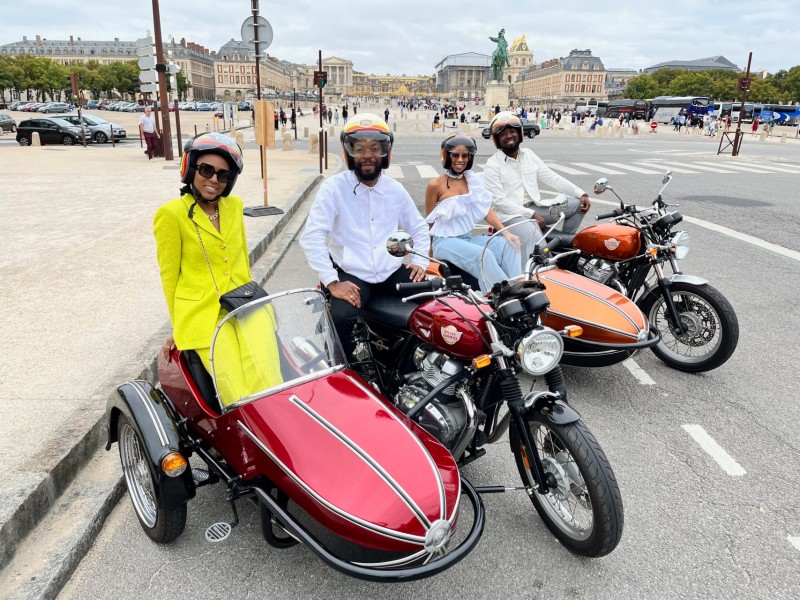In the foreground of the image, we see four people posed cheerfully for a picture. The setup features two motorcycles, each equipped with a sidecar. On the left, a black woman dressed in a bright yellow suit with a black purse and large black sunglasses is seated in a shiny red sidecar. The red motorcycle attached to this sidecar is ridden by a black man wearing a white shirt, black pants, and a helmet with vibrant red, yellow, and orange details. He has a black beard and gold rings on his fingers. 

To the man's right, another black woman is perched in an orange sidecar, wearing a white one-shoulder frilly top and blue jeans, her helmet visor up. Beside her, another black man with a black beard, dressed in a white shirt and gray pants, rides the orange motorcycle with similar black detailing. 

In the background, a historical and bustling European setting unfolds. The architecture is classical, featuring an ornate government building and a prominent horse statue. People and cars fill the scene, indicating a lively, heavily toured area. The sky above is slightly cloudy yet retains a hint of blue, giving the entire scene a cozy, modern-day feel.